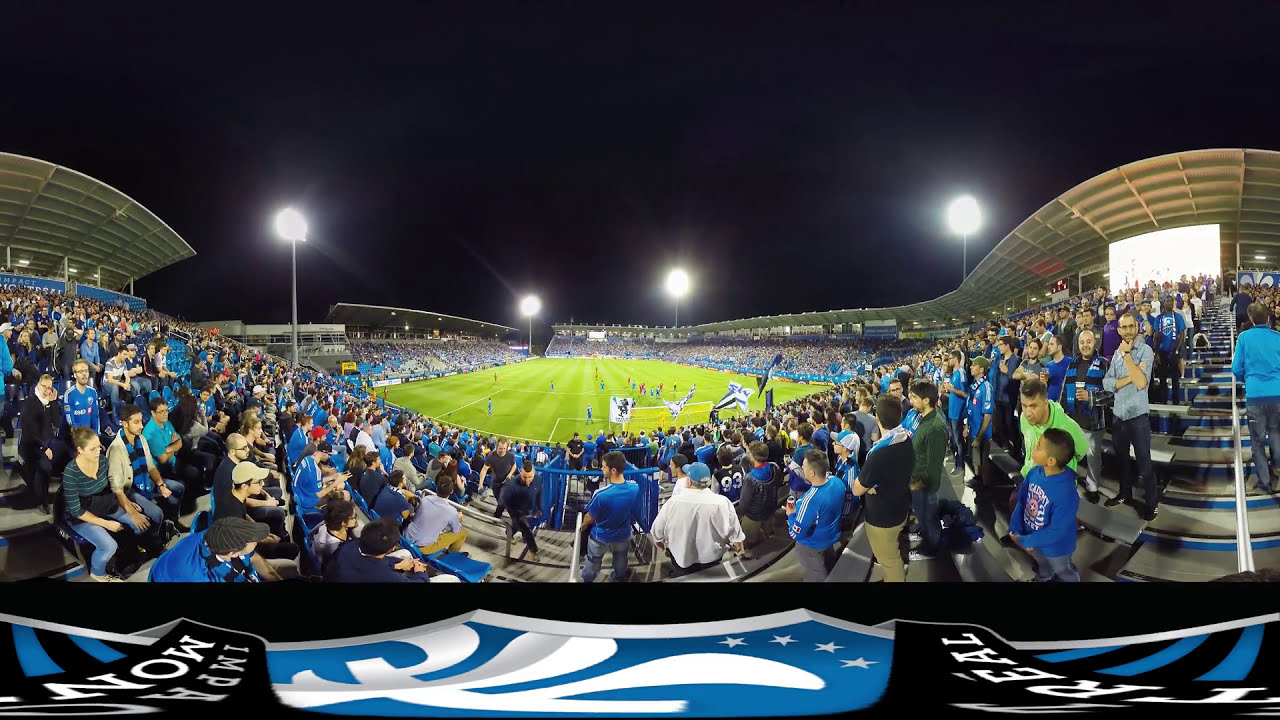The image captures a dynamic nighttime soccer game at a packed Montreal Impact home stadium, taken from a high vantage point behind one of the goals with a 360-degree camera. The scene is vibrant with fans, predominantly dressed in blue, energetically supporting their team. The vast green pitch, marked with white lines, hosts players from the blue-clad home team and their red-uniformed opponents. Towering stadium lights illuminate the field under a pitch-black sky. The curved overhang of the stadium is visible to the sides, and the stands are filled with cheering spectators, creating a wave-like effect around the edges of the image. The Montreal Impact logo and banners are prominently displayed, adding to the electrifying atmosphere of this thrilling night game.